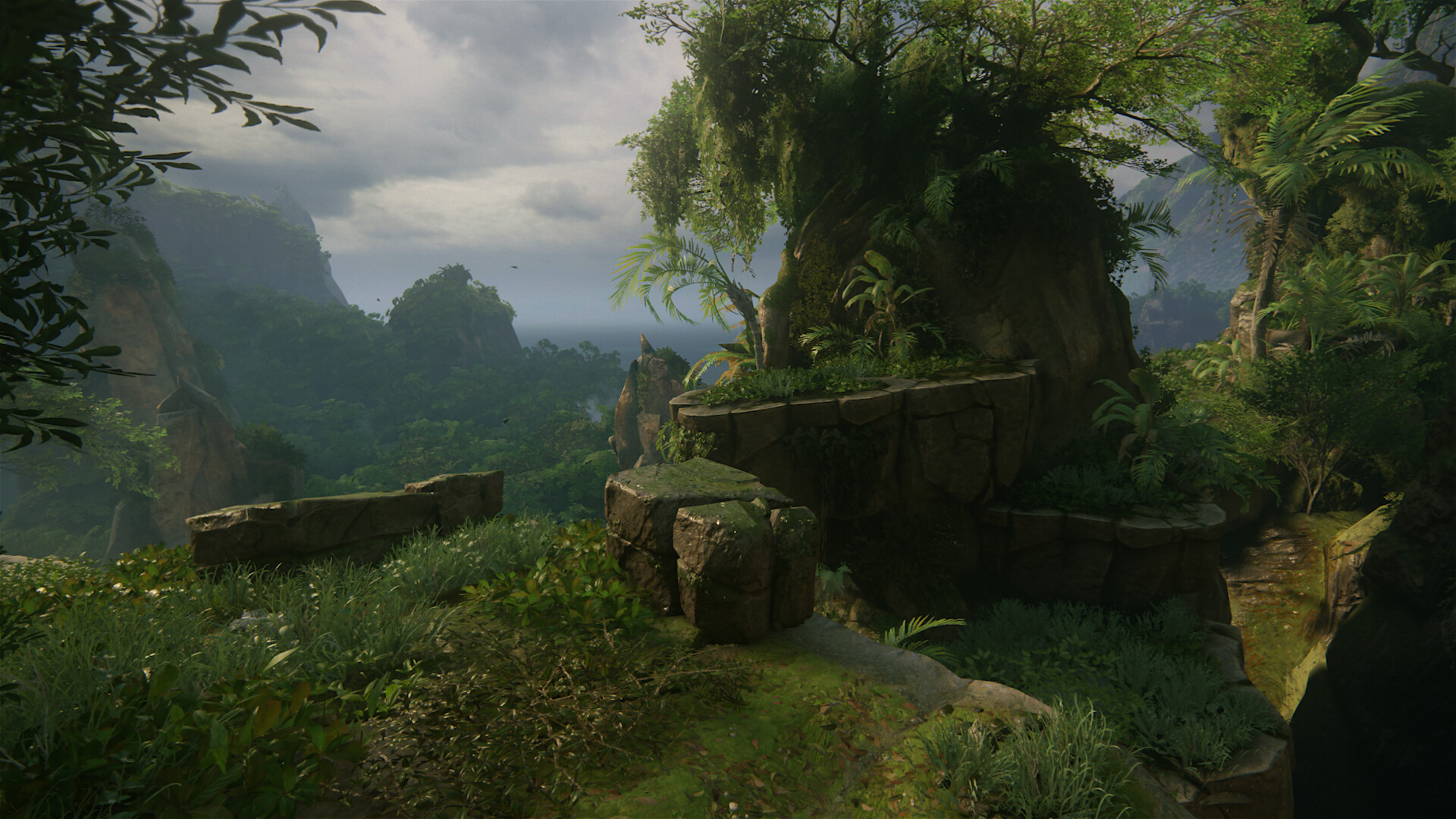A stunning piece of outdoor concept art portrays an ancient, overgrown ruin nestled in a lush, jungle-like environment. The scene is dominated by thick, verdant grass and large, flourishing leaves. In the foreground, a half wall of rocks hints at the remnants of former structures, now reclaimed by nature. Towering trees, including majestic palm trees, with their vast palm leaves, contribute to the dense greenery. To the right of the image, patches of exposed dirt break the continuity of the flora. The backdrop features a towering mountain bathed in the soft glow of a blue sky, partly obscured by dramatic, cloudy skies. Amidst the vibrant scene, birds can be spotted soaring around the grassy mountain in the distance, adding life to this serene, forgotten world.